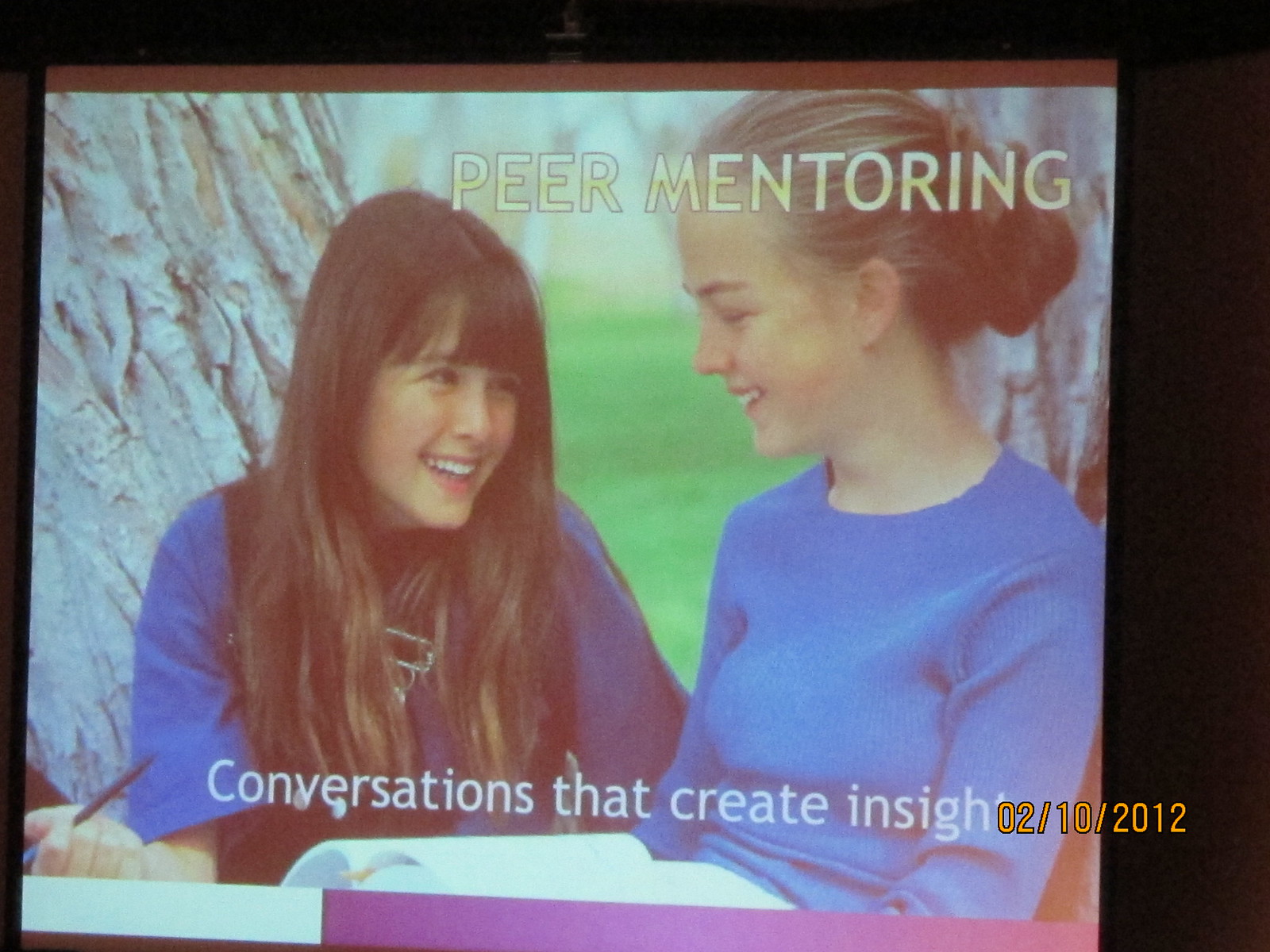The image captures a photograph displayed on a monitor or TV screen, bordered by a black frame. The central scene features two teenage girls sitting outside by a grassy field, flanked by trees. The girl on the left has long brown hair cascading past her shoulders, is of Asian descent, and wears a blue t-shirt. She smiles warmly at the blonde girl on the right, who has her hair pulled back into a bun and is also dressed in a blue shirt. An open book rests on the blonde girl’s lap as they share a moment of conversation and smiles. At the top of the image, in yellow text, it reads "Peer Mentoring," while white text at the bottom declares "Conversations That Create Insight." A timestamp on the bottom right corner marks the date as 02/10/2012.